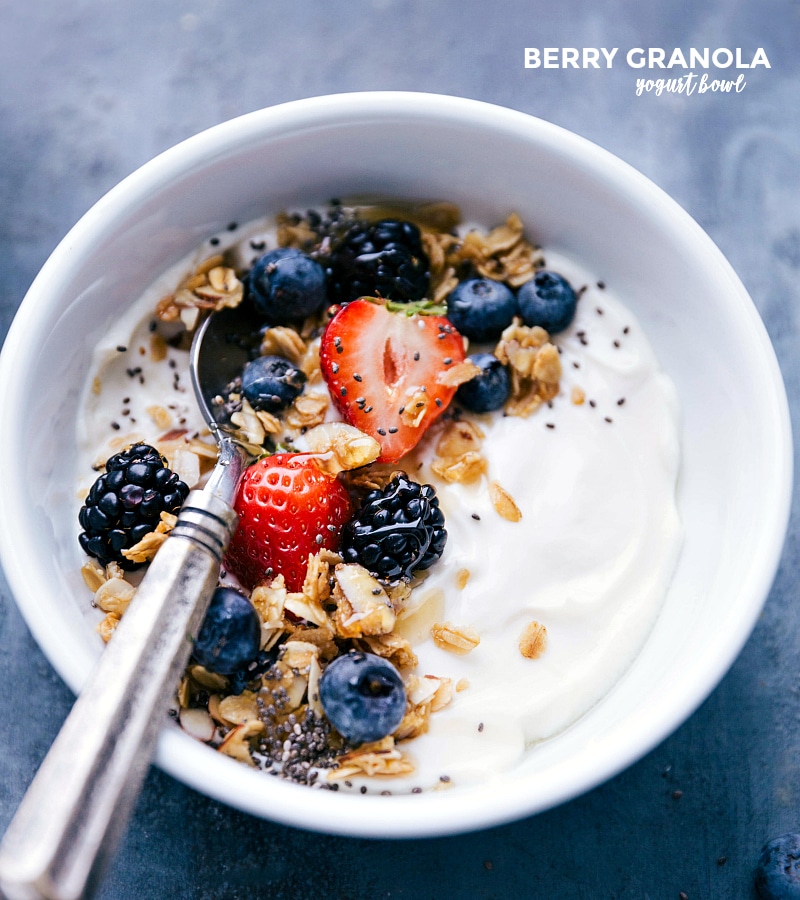This is a detailed product image featuring a Berry Granola Yogurt Bowl, likely intended for an advertisement or a recipe guide. The photograph, taken from an overhead perspective, showcases a white bowl placed on a dark blue surface. The bowl is filled with white, unflavored yogurt and an assortment of toppings, including granola flakes, chia seeds, blueberries, blackberries, and two strawberries. The toppings are predominantly positioned on one side of the bowl, while the other side remains plain. A silver spoon is inserted into the side of the bowl that has granola and blueberries. In the top right-hand corner of the image, the text "Berry Granola Yogurt Bowl" is written in cursive. The clean and vibrant presentation highlights the freshness and variety of the ingredients, making it an enticing option for a healthy meal or snack.